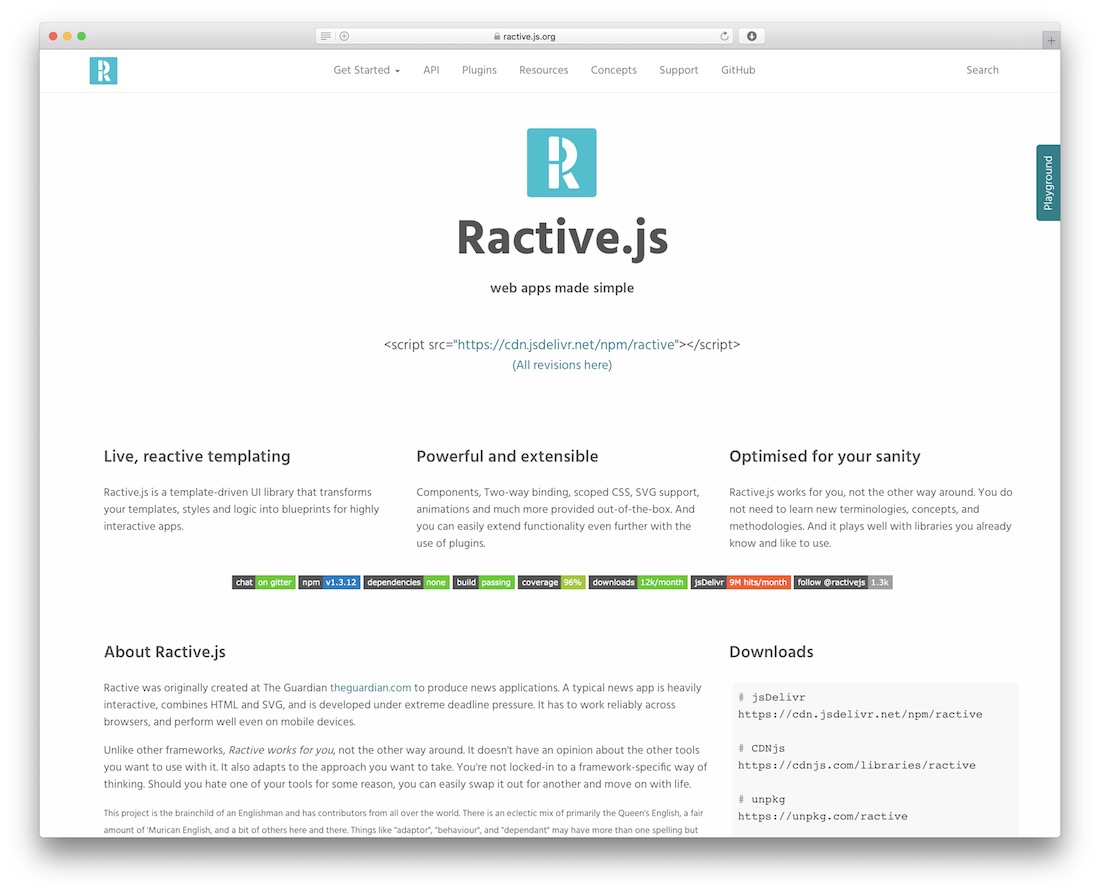The website features a distinct green box in the upper left-hand corner with a disjointed white "R" emblem. This represents "Reactive.js," with the tagline, "Web Apps Made Simple." At the top of the page, the URL reads "reactive.js.org," and a navigation bar offers options such as "Get Started," "API," "Plugins," "Resources," "Concept," "Support," and "GitHub." In the upper right-hand corner, a search bar is also available.

Central to the webpage, there is a script address link, suggesting that all revisions can be accessed there. On the right side, a box labeled "Playground" invites users to experiment with the framework directly on the site. 

The webpage content is organized into paragraphs presenting key features: "Live Reactive Templating," "Powerful and Extensible," and "Optimized for Your Sanity," each described in further detail. Additionally, a visually striking bar with colorful segments—black, green, blue, and red—features white writing and stretches across the page. Further down, a section elaborates on Reactive.js through a series of paragraphs and provides download links within a gray box.